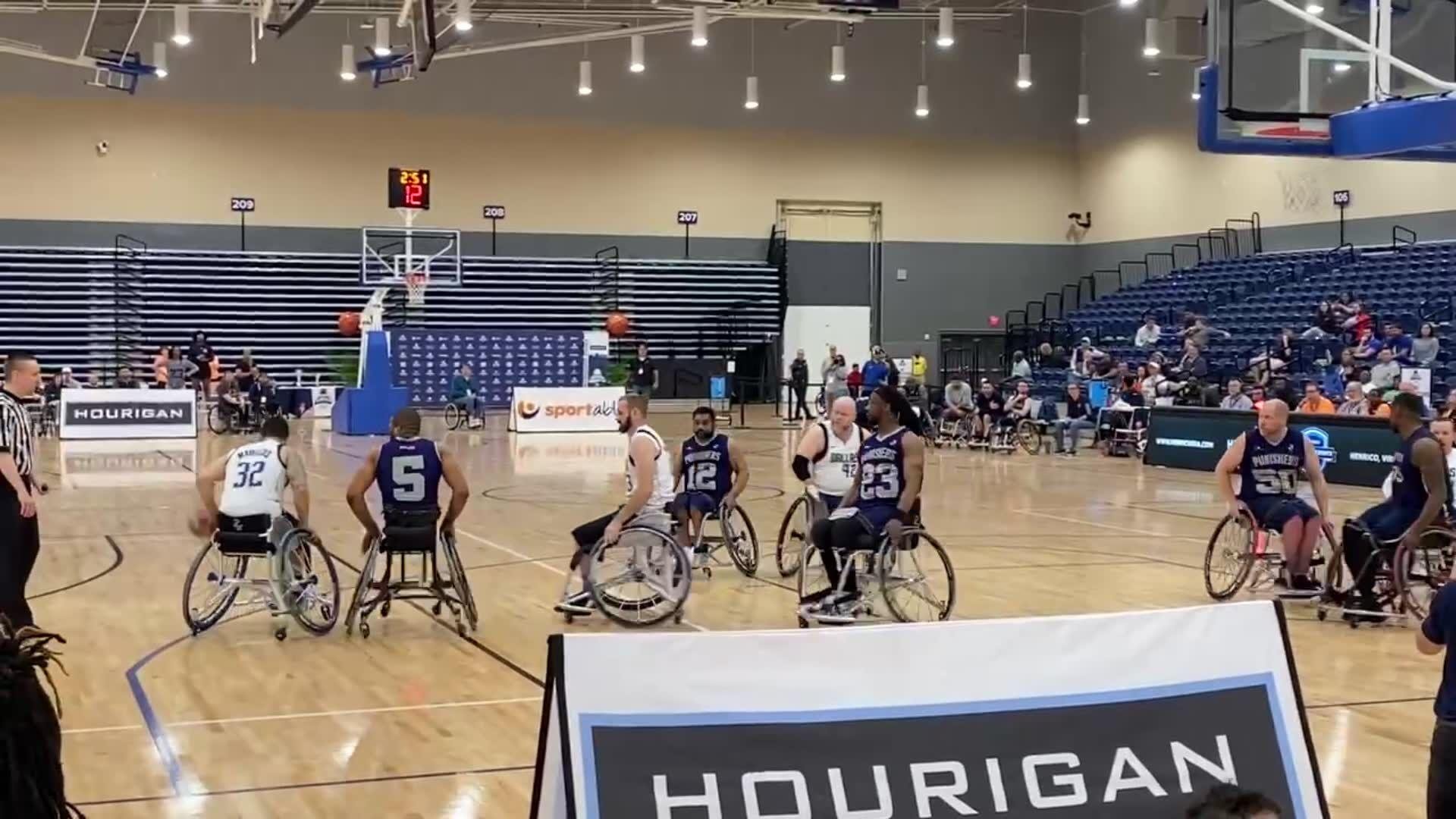The photograph captures an intense wheelchair basketball game inside a small gym, possibly a high school gymnasium. The gym features hanging white lights from the ceiling and mostly empty blue bleachers in the background, with some spectators seated towards the front. The shiny hardwood court, marked by tape delineating different sections, hosts two three-on-three teams. One team is dressed in dark navy jerseys with large gray numbers, while the opposing team wears white jerseys paired with dark shorts and dark lettering. Two referees are visible; one is positioned on the far left in a black and white striped top and black trousers. White signs are strategically placed around the court, acting as barriers, including a prominently featured banner reading "H-O-U-R-I-G-A-N" in the foreground. A scoreboard in the background reads "2.51" and "12" in red, adding to the competitive atmosphere of the game.